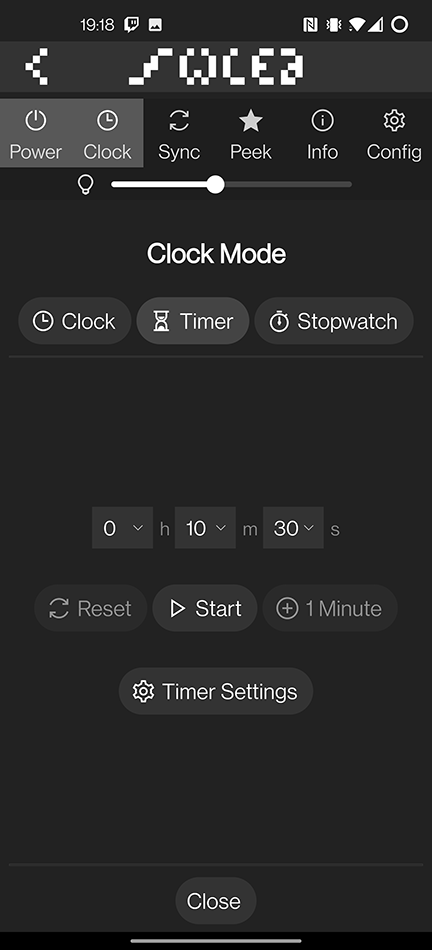The image shows a mobile application interface displayed in dark mode, designed as an all-in-one clock utility. The app's name appears at the top in a low-resolution, charming 8-bit font, likely spelling "S-O-L-E-A" or a similar variation. The interface features several menu options, including Power, Clock, Sync, Peak, Info, Configuration, and Brightness Settings. In the lower section, the app presents various modes such as Clock, Timer, and Stopwatch, with the Timer mode currently active and set to 10 minutes and 30 seconds. To operate the timer, there are clearly visible Start, Reset, and Add One Minute buttons. At the very bottom, additional Timer Settings and a Close button can be found. All text elements are rendered in white, enhancing readability against the dark background.